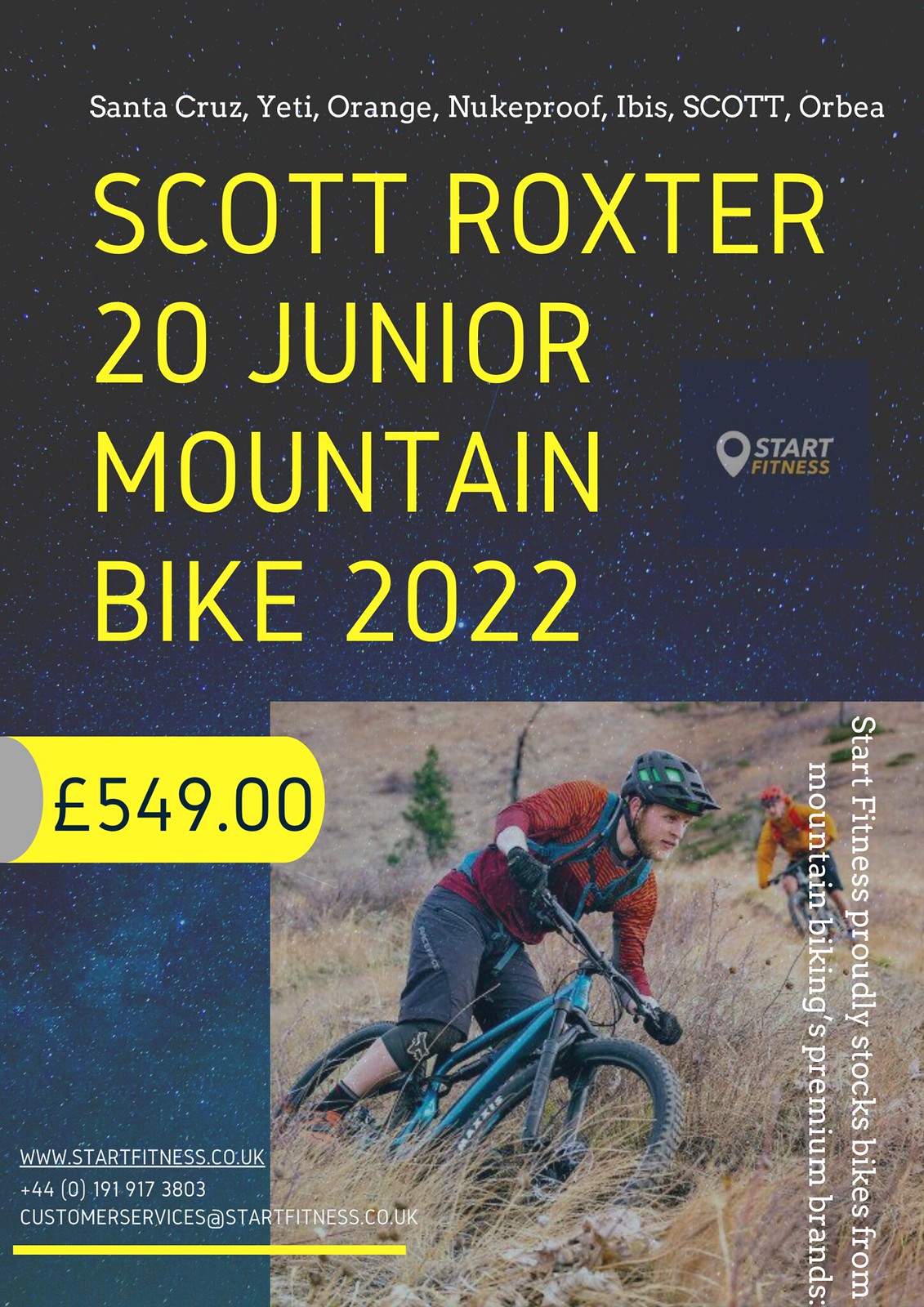The image appears to be the cover of a magazine or an advertisement, predominantly dark blue with white dots that lighten toward the bottom. At the top, the brand names "Santa Cruz," "Yeti," "Orange," "Nukeproof," "Ibis," "Scott," and "Orbea" are listed in white text. Centered prominently in large yellow letters is the title "Scott Rockster 20 Jr. Mountain Bike 2022." A bright yellow tab on the side indicates the price as £549.00. 

In the lower right corner of the cover, there is a depiction of two bike riders. The closer cyclist is wearing a black helmet, a red shirt, and shorts, while riding a blue bike through a field of beige dry grass, slightly leaning to the side. Another cyclist, dressed in an orange outfit, is visible in the far distance. Both riders are wearing helmets. The bottom left corner includes the text: "Start Fitness proudly stocks bikes from Mountain Biking's premium brands," along with a website URL, www.startfitness.co.uk.